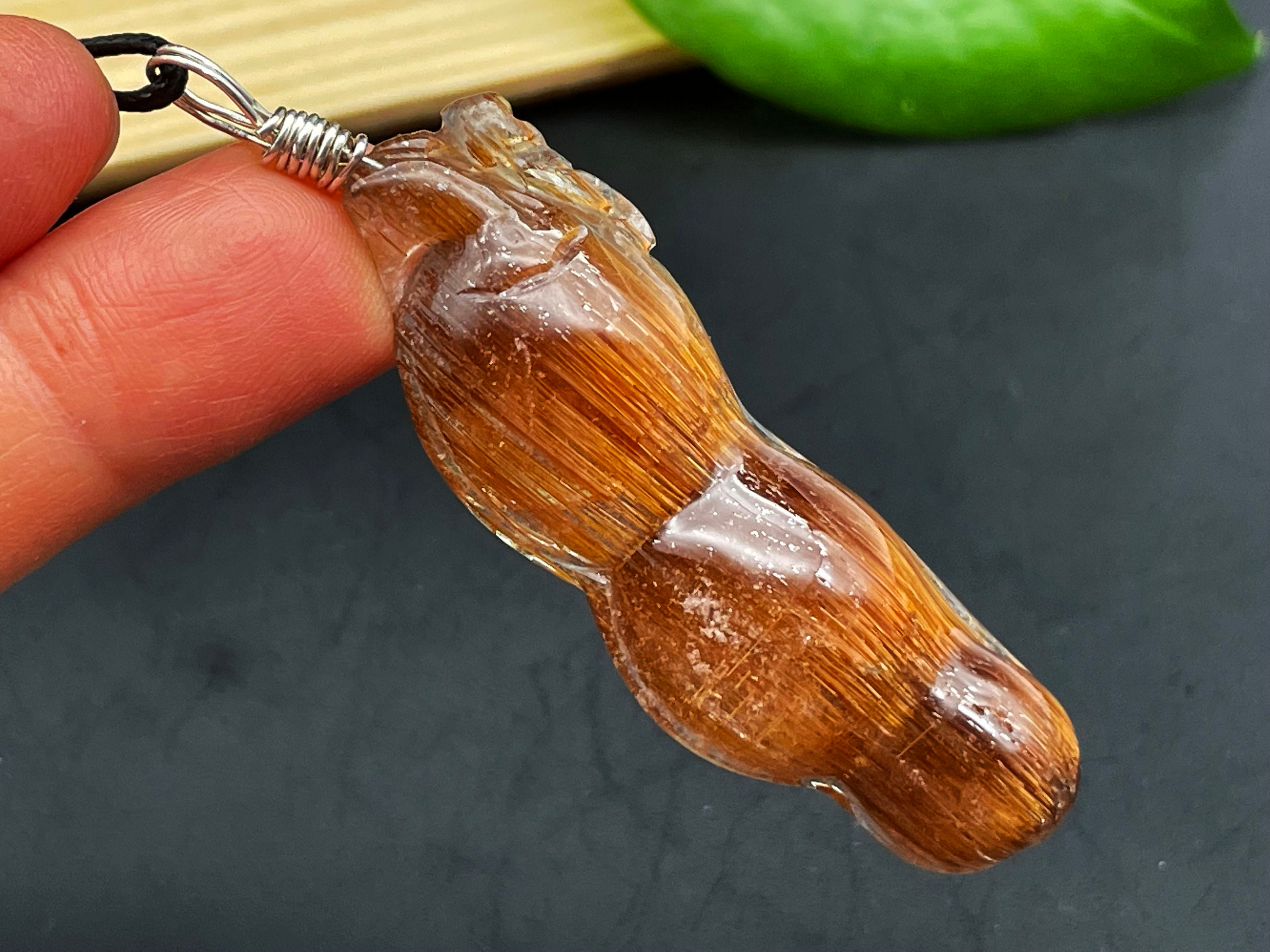This photograph features a close-up view of a person holding a small, intricately crafted item between their fingers, prominently positioned in the upper right corner of the image. The item appears to be a beautifully textured piece of petrified wood encased in clear resin, designed to resemble a stack of three vertically arranged pumpkins or possibly a ginseng-like form segmented into three parts. The detailed woodwork is encased within a thick, smooth resin, creating a clear, glossy surface. Thin fibers and carved textures are visible within, giving the object a unique and artistic appearance. A metal hook is attached to the top of the resin, connecting the piece to a rope or chain, suggesting it is intended to be worn as a pendant or keychain. The background of the photograph includes a hint of green at the top, likely a leaf or the corner of a cutting board, set against a dark gray table. The close-up nature of the image emphasizes the craftsmanship and distinctive characteristics of the item, making it a focal point against the subdued backdrop.